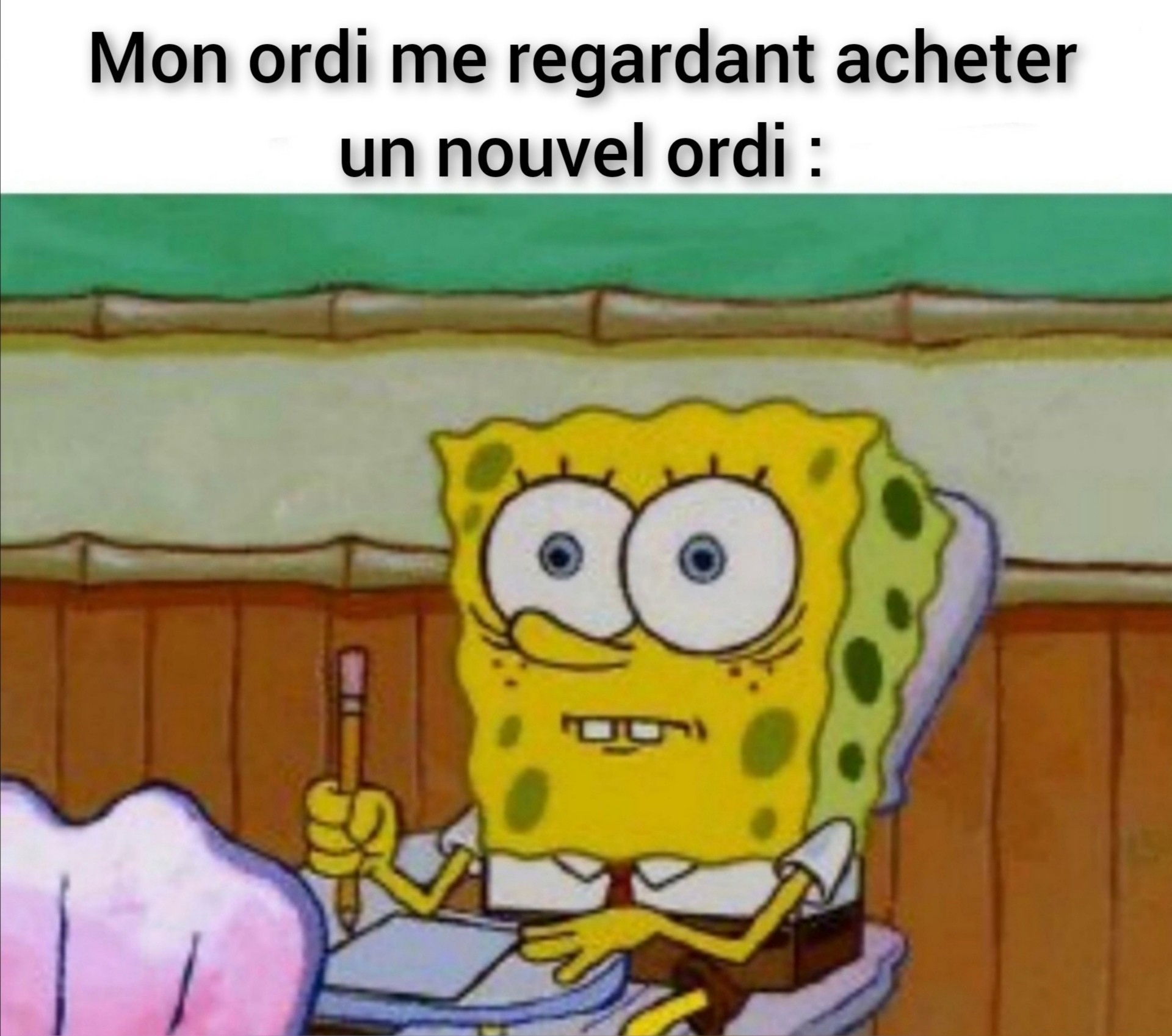The image is a meme featuring Spongebob Squarepants, set in a driving school classroom. Spongebob is seated at a desk, gripping a pencil in his right hand with a paper in front of him. He is depicted with a highly worried and shocked expression, characterized by his large, wide eyes. The background showcases wood paneling on the lower portion, a strip of white wainscoting, and an old-fashioned green chalkboard. Partially visible in front of him is the seashell-shaped seat. The meme has black text at the top written in French, reading "mon ordi, me regardant acheter un nouvel ordi," which translates to "my computer, watching me buy a new computer." The text is on a white background, and the meme image itself is a screenshot from a Spongebob episode.